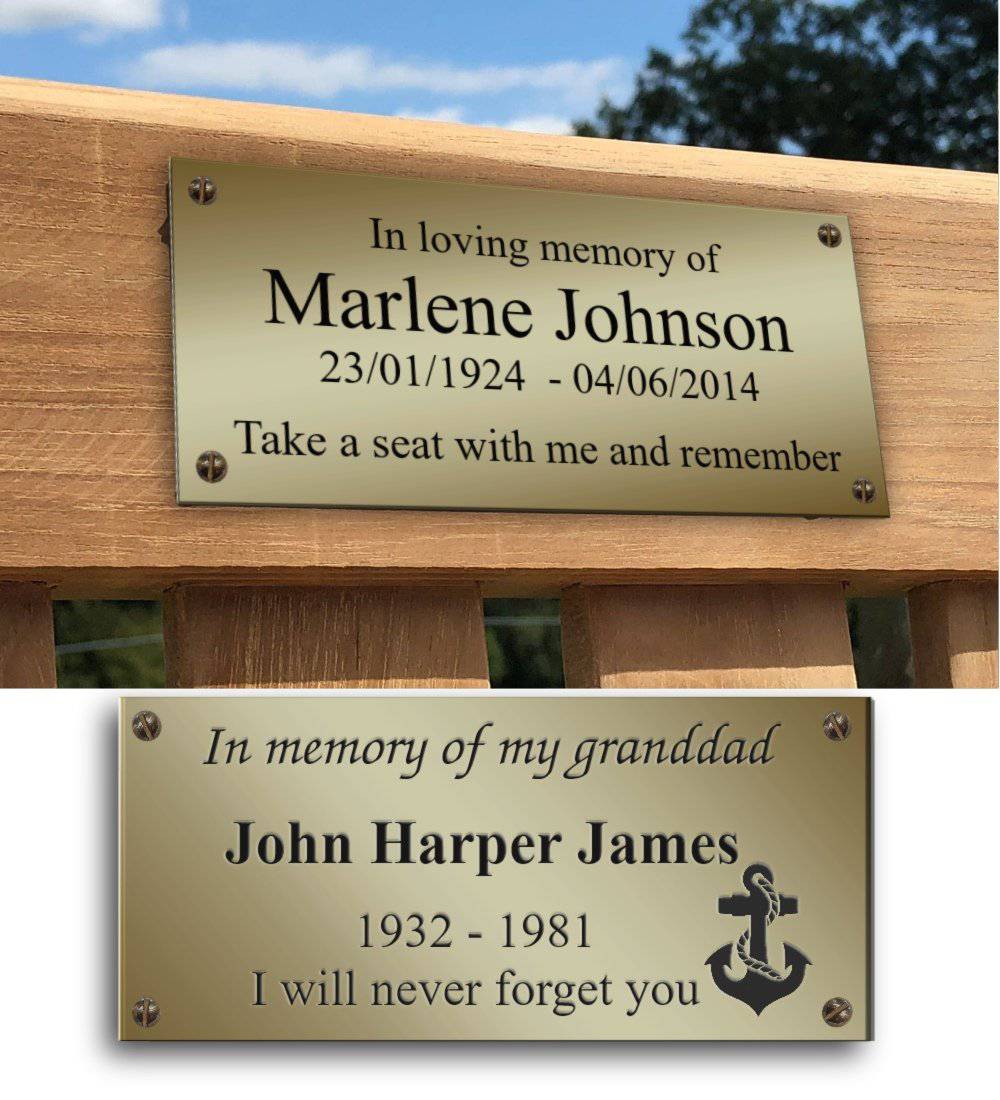The image features two detailed, metallic plaques, each framed separately. The top part of the frame showcases a rectangular bronze-colored plaque mounted on a light-colored wooden surface, likely a park bench. The plaque, accompanied by a backdrop of blue skies, clouds, and distant trees, reads: "In loving memory of Marlene Johnson" with the dates "23-01-1924 to 04-06-2014." Below, it states, "Take a seat with me and remember."

The bottom part of the frame displays another similarly metallic plaque, not affixed to anything. It features the message: "In memory of my granddad," italicized, followed by "John Harper James," in bold, with the dates "1932-1981" beneath. The plaque concludes with the tribute, "I will never forget you," and is adorned with an anchor and rope, hinting at a Naval connection for John Harper James.